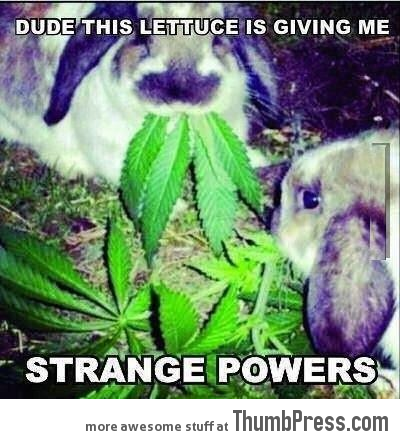This square image, designed as a meme, features a humorous scene with two rabbits in a grassy area. The rabbit situated at the top left faces forward, displaying predominantly white fur with some brown markings, a black snout, and black ears. This bunny is munching on three bright green, long leaves, which resemble marijuana leaves, sticking out of its mouth. Another rabbit is seen emerging from the right side of the image, showing its left profile with similar white and brown fur, a black and white ear, and a large, visible eye. Scattered on the ground are more of these green leaves. The text within the image reads, "DUDE, THIS LETTUCE IS GIVING ME" in large white font at the top, and "STRANGE POWERS" in white, outlined black, all-caps letters at the bottom. Beneath the image, there is a watermark stating "more awesome stuff at ThumbPress.com."